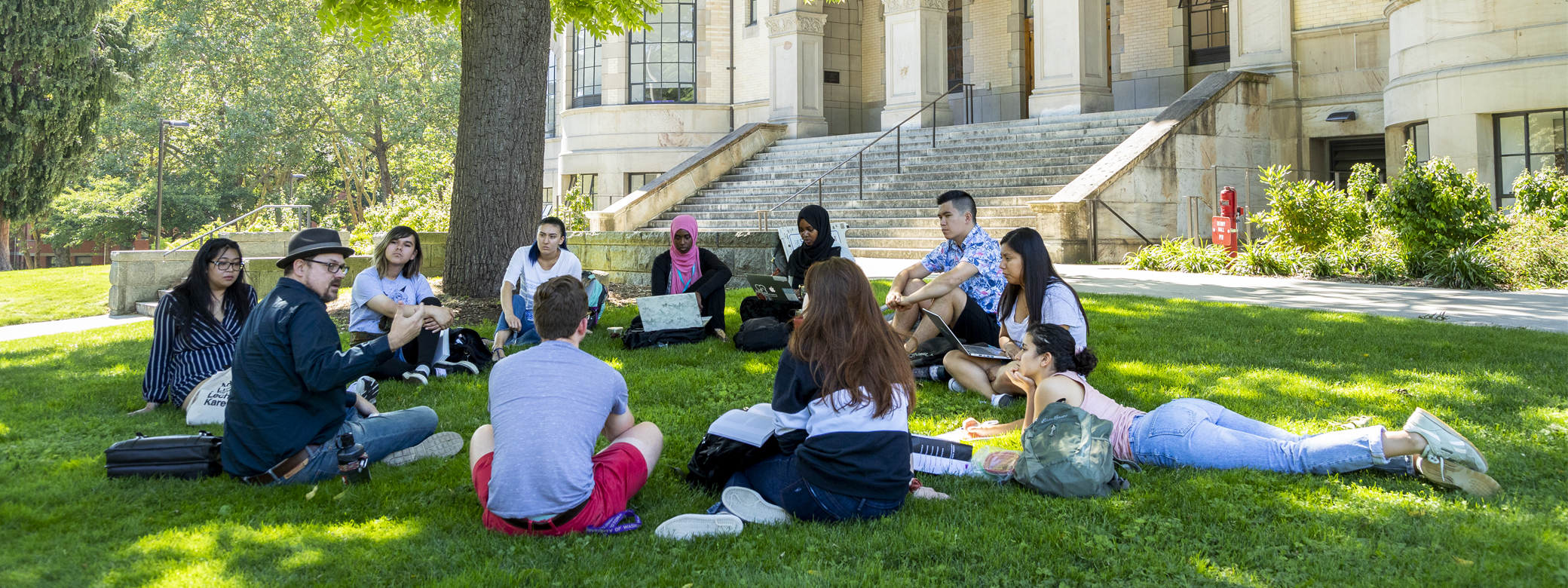The image depicts a lively outdoor study session with a group of twelve students seated in a circle on a lush, green lawn, likely on a college campus. They are positioned in front of a whitish-beige building with concrete steps, suggesting it could be a school or university building. The scene is framed by vibrant greenery, including a prominent tree in the middle ground and a glimpse of a small forested area in the background. 

The students appear to be college-aged and are engrossed in their laptops, engaging in what seems to be a collaborative project or study group. One individual, possibly an older professor or teacher, stands out among them. Positioned on the left side of the image, he is wearing glasses, a hat, a dark shirt, and jeans, and appears to be leading the discussion, capturing the attention of the group. 

Notably, there is a girl lying on her stomach with her legs stretched out, indicating a casual and relaxed atmosphere. The setting suggests springtime, with the grass and trees in full, vibrant bloom, and there's even a fire hydrant visible in the background for an added touch of campus detail.